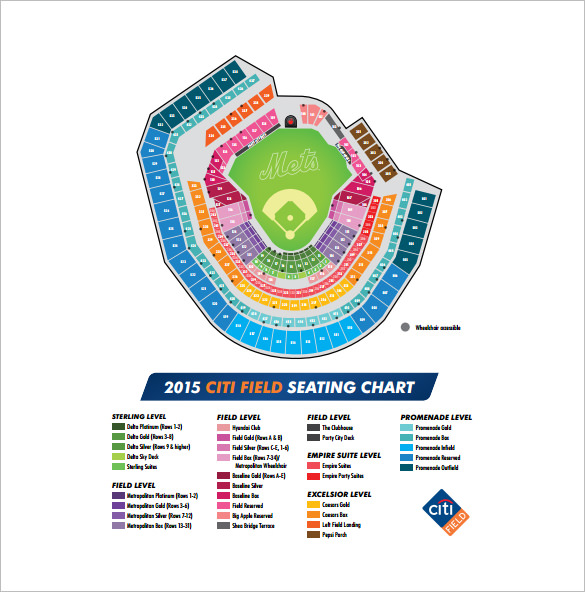A detailed seating chart of a stadium, presented with a clean, white background and bordered by a thin, light gray line. The focal point of the image is a green baseball field with a clearly visible diamond at the center, displaying the word "Mets." The seating arrangement is depicted with varying colors: the outermost seats are blue, followed by rows of teal green, then yellow, and finally red. The seats closest to the field are grouped in colors of purple, pink, and green. 

Below the seating visualization is a blue rectangle featuring the text "2015" in white, and "CITI FIELD" in orange, followed by "seating chart" in white. The bottom portion of the image includes four columns, each serving as a legend for the seating chart. Each column lists differently colored rectangles representing distinct seating areas, accompanied by descriptions and row numbers printed in very small, almost unreadable text. At the bottom of the rightmost column is the CITI Field logo.